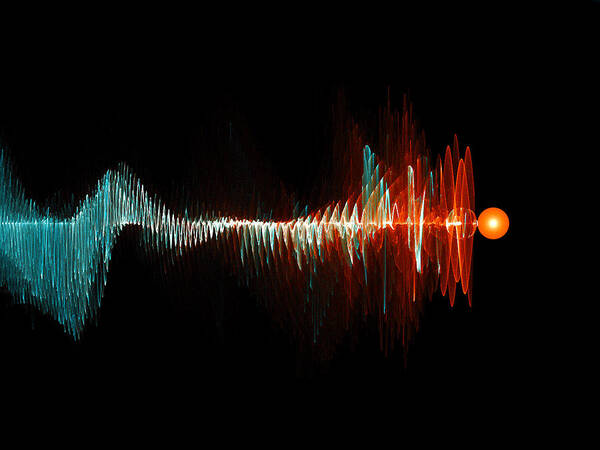The image features a dynamic and visually compelling depiction of particle-wave duality on a black background. Dominating the scene is a series of vividly colored waves and circles that convey a 3D effect. At the center-right is a small, vibrant orange ball with a white outline next to it, illustrating the particle aspect. Extending from this ball are undulating red wavelengths, which evoke the impression of sound waves or energy radiating outward. These red waves mix subtly with light blue hues, transitioning through to dark blue as they extend further from the orange ball. The blue waves grow increasingly tight and small, culminating near the lower left in a triangular shape. A distinct white line runs through the center of the composition, originating from the orange ball, reinforcing the interconnectedness of the depicted phenomena. The overall effect is a striking visual representation of the interplay between particle and wave forms.